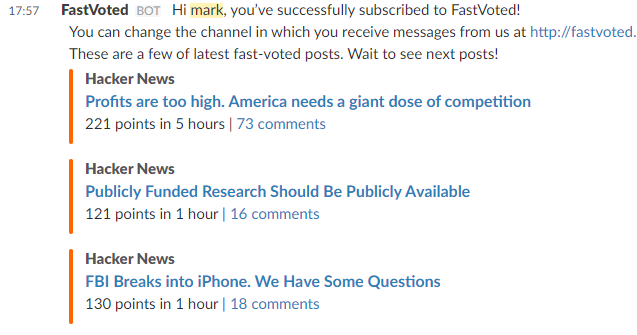At 5:57 p.m., the image features a pristine white background with bold black text that reads: "Fast Voted Bot." The message begins with a greeting, "Hi Mark," where the name "Mark" is highlighted in yellow. The text continues, informing Mark that he has successfully subscribed to Fast Voted. It offers the option to change the channel for receiving messages at http://fastvoted.com. Below this, the image displays recent Fast Voted posts in a vertical arrangement, marked by an orange line running parallel to the posts. 

The first post is from Hacker News, titled "Profits are too high. America needs a giant dose of competition," garnering 221 points in five hours and receiving 73 comments. The second post, also from Hacker News, asserts that "Publicly funded research should be publicly available," which has achieved 121 points in one hour along with 16 comments. The third post, another Hacker News entry, is titled "FBI breaks into iPhone. We have some questions," accumulating 130 points in one hour with 18 comments. This is the entirety of the displayed content in the image.